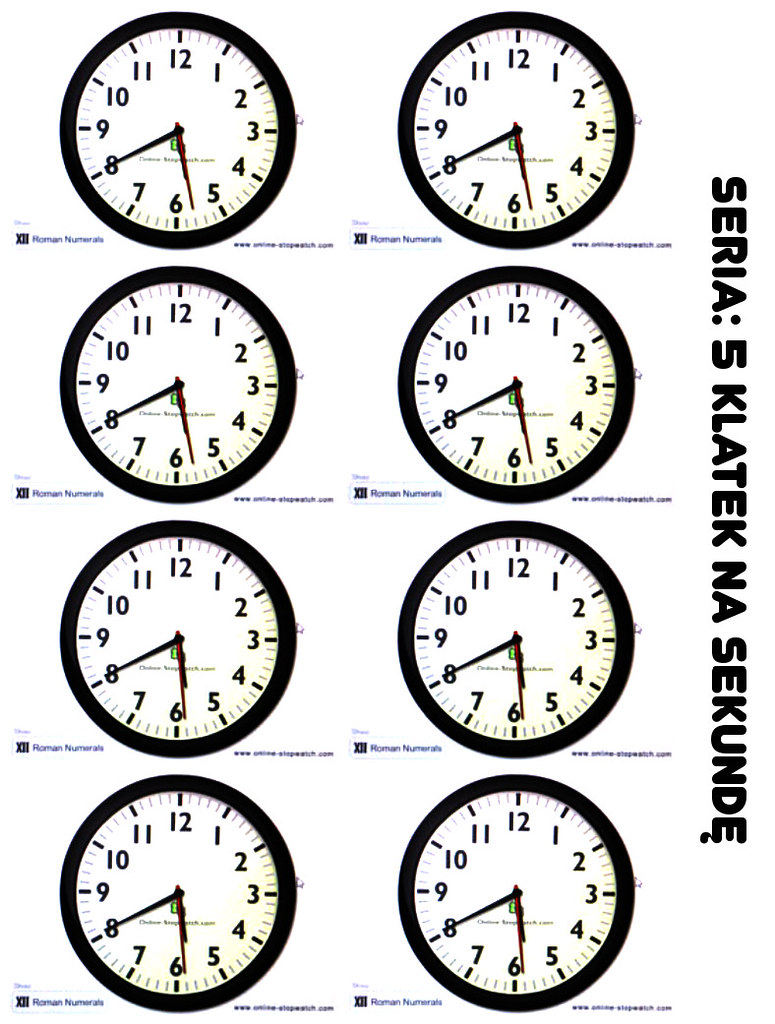The image features a printable chart on a white background, showcasing a grid of eight computer-generated, black-framed clocks arranged in two rows of four vertical clocks each. Each clock has a black face with black numerals and shows the exact same time, 5:40, with the red second hand positioned just before the six, aligned with the hour hand. Small black writing is present at the bottom left and right corners of each clock face, suggesting they can be individually cut out. To the side of the page, written vertically, are the words "Syria 5 Clatic na Secunda" in a language other than English. This appears to be a poster or advertisement, potentially for this specific clock brand.